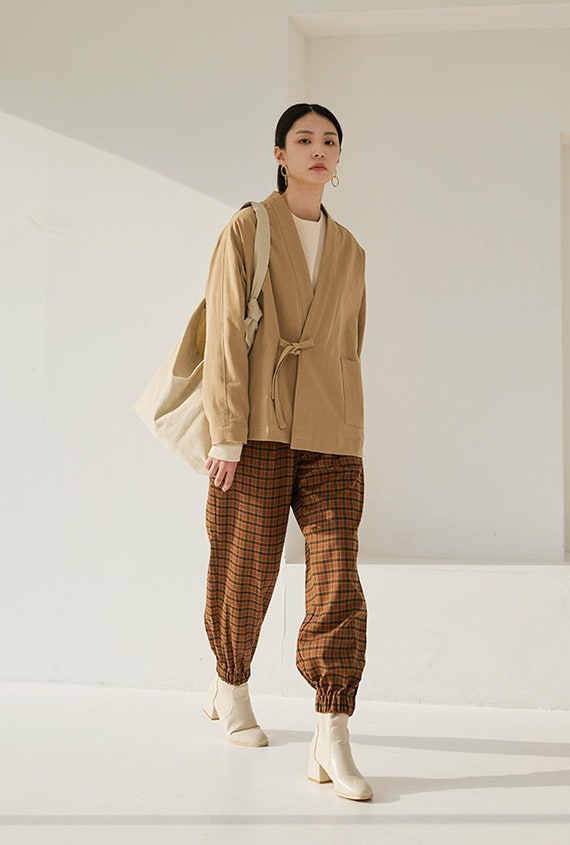A young and elegant Asian woman, possibly in her late 20s or early 30s, is confidently walking towards the camera in a professional modeling photograph. Set against a crisp white background with excellent lighting, she makes direct eye contact with the lens. Her dark hair is neatly pulled back into a ponytail, accentuating her red lipstick and small gold hoop earrings. Dressed in a stylish and coordinated outfit, she wears a white shirt partially visible under a light brown cardigan tied in the front. She carries an off-white fabric bag on her right shoulder and sports black and brown checkered pants with elastic at the ankles. Her outfit is rounded off by large white boots that peek out from under her pants. The image showcases a harmonious blend of neutral colors, including various shades of tan, brown, black, and white. The woman’s poised demeanor and sophisticated attire make her the focal point of this visually striking and professional photograph.